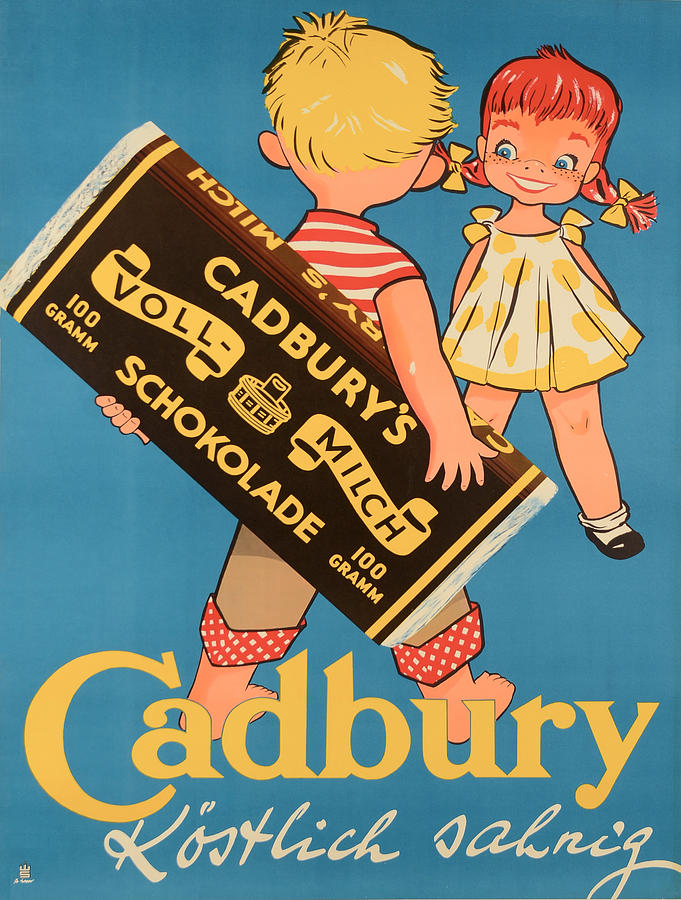This vibrant vintage-style cartoon advertisement for Cadbury's chocolate features two charming, cartoonish children. The scene portrays a boy with his back to us, concealing a giant chocolate bar behind him. The bar is prominently brown, adorned with yellow lettering and stripes displaying the name "Cadbury's." Opposite him, a smiling girl with pigtails stands facing the boy, dressed in a cheerful yellow and white dress. The ad is set against a lively blue background, which contrasts beautifully with the characters' bright outfits.

At the top of the chocolate bar, a banner unfolds with text in a European language, reading "V-O-L-L" and "M-I-L-C-H," suggesting it's for Cadbury's milk chocolate. Below, the phrase "100 gram with two M's" is visible, likely indicating the weight of the chocolate bar in metric measurements. Positioned at the bottom of the advertisement, the word "Cadbury" is prominently displayed in bold yellow letters, accompanied by cursive script in white, also in the non-English language. The overall effect is both nostalgic and eye-catching, drawing attention to the timeless allure of Cadbury's chocolate.